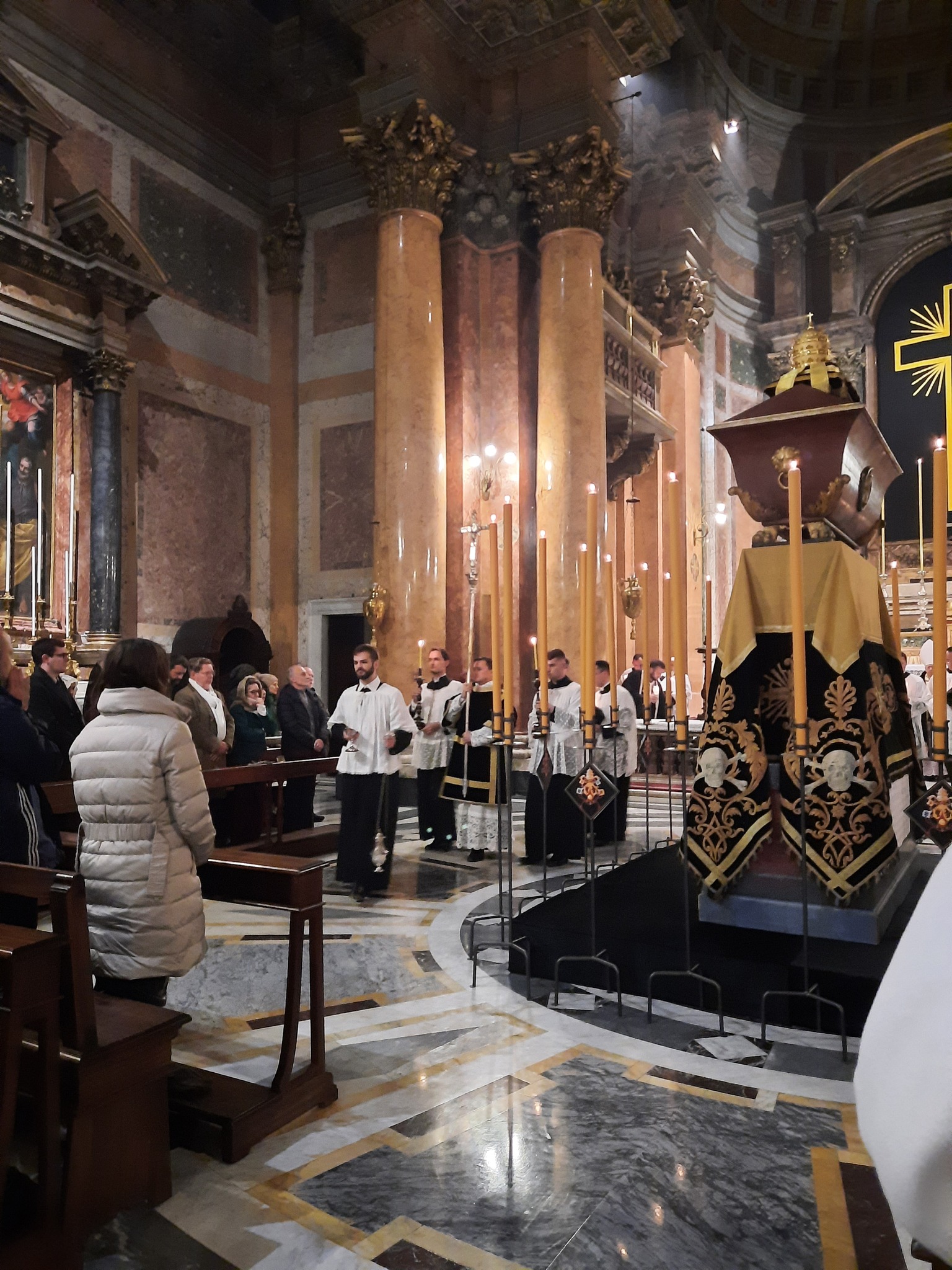This photograph captures an ornate and grand Catholic cathedral during a solemn Mass or funeral. The view is from the rear of the congregation, showcasing a procession of clergymen moving towards the altar. The men, dressed in intricate black robes with white tops, carry tall candles and a large cross. One of the men in front is holding a chalice. The church is bustling with worshippers wearing coats, lined along the pews to the left.

The cathedral is visually striking with its majestic, peach marble columns topped with acanthus leaves and a floor of gray marble squares adorned with brown and gold motifs. Central to the image is a prominent, elevated monument surrounded by at least twelve lit candles. This monument, possibly a casket or sarcophagus, is set on an elaborate gold and black filigree-style rug featuring skull and crossbones. The altar beneath it is draped in matching gold and black cloth. The overall scene is one of reverent grandeur, accentuated by the structure’s elaborate columns and ornate marble floors.